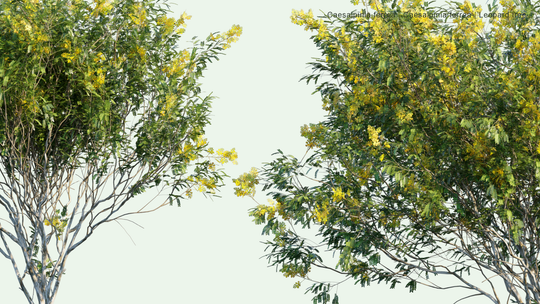The horizontally aligned, rectangular photograph captures a serene, upward view of a hazy light blue sky framed by two trees. On the left, a slender tree with a thin trunk extends an intricate network of branches, each adorned with a mix of green, light green, and yellow leaves that create a graceful, airy impression. The right side is dominated by a denser tree, its branches brimming with a blend of green and yellow foliage, some mixed in with small, yellow flowers that resemble forsythia blooms. Despite the hazy sky and slightly obstructed tiny printed text in the upper right corner, the vivid greenery and subtle hues of yellow flowers create a tranquil and picturesque scene.